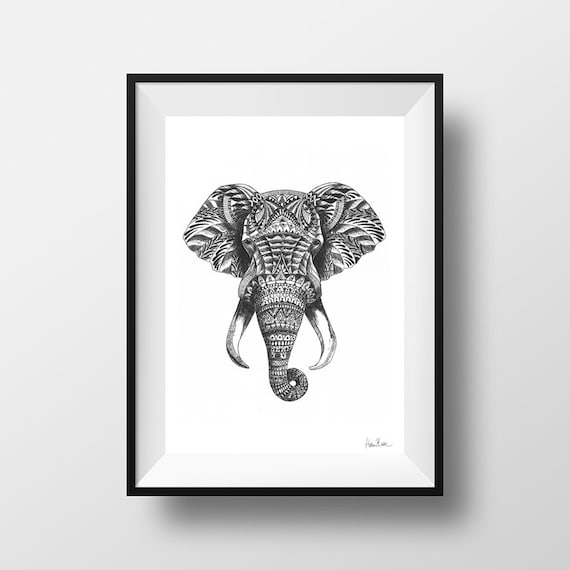This photograph depicts a framed black-and-white illustration of an elephant's head and tusks, set against a white background. The elephant's skin is intricately adorned with tribal designs, styled like tattoos that swirl over the ears and face, incorporating geometric shapes, zigzag patterns, and striped designs. The elephant's two white tusks are prominently featured, and a small cursive signature is visible in the bottom right corner of the artwork. The simple frame, which is about an inch thick, creates a shadow on the white wall, suggesting it protrudes slightly. The artwork is highly detailed, combining the realistic form of an elephant with abstract, graffiti-like textures to replace its natural skin, creating an elaborate and unique visual effect.